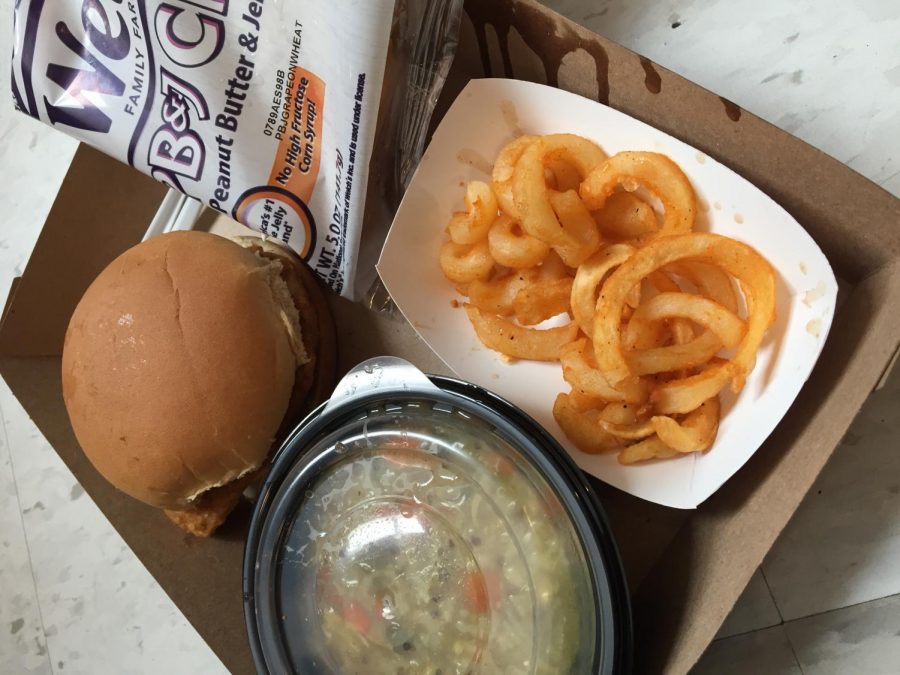This image depicts an overhead view of a simple, fast food lunch served in a brown cardboard tray, possibly intended for a schoolchild. The tray contains a smaller white cardboard container filled with golden deep-fried curly fries. Adjacent to it is a black plastic bowl with a clear lid, housing what appears to be chicken noodle soup with visible chunks of carrot, pasta, and chicken broth. In the top left corner of the tray sits a hamburger bun encasing what seems to be a fried chicken patty, though the exact specifics are unclear. Additionally, there is a partially visible plastic bag with an orange banner that appears to label the contents as a peanut butter and jelly product, prominently highlighting that it contains no high fructose corn syrup. The tray is placed on what looks like a white tile surface, suggesting an informal setting like a cafeteria or school environment.